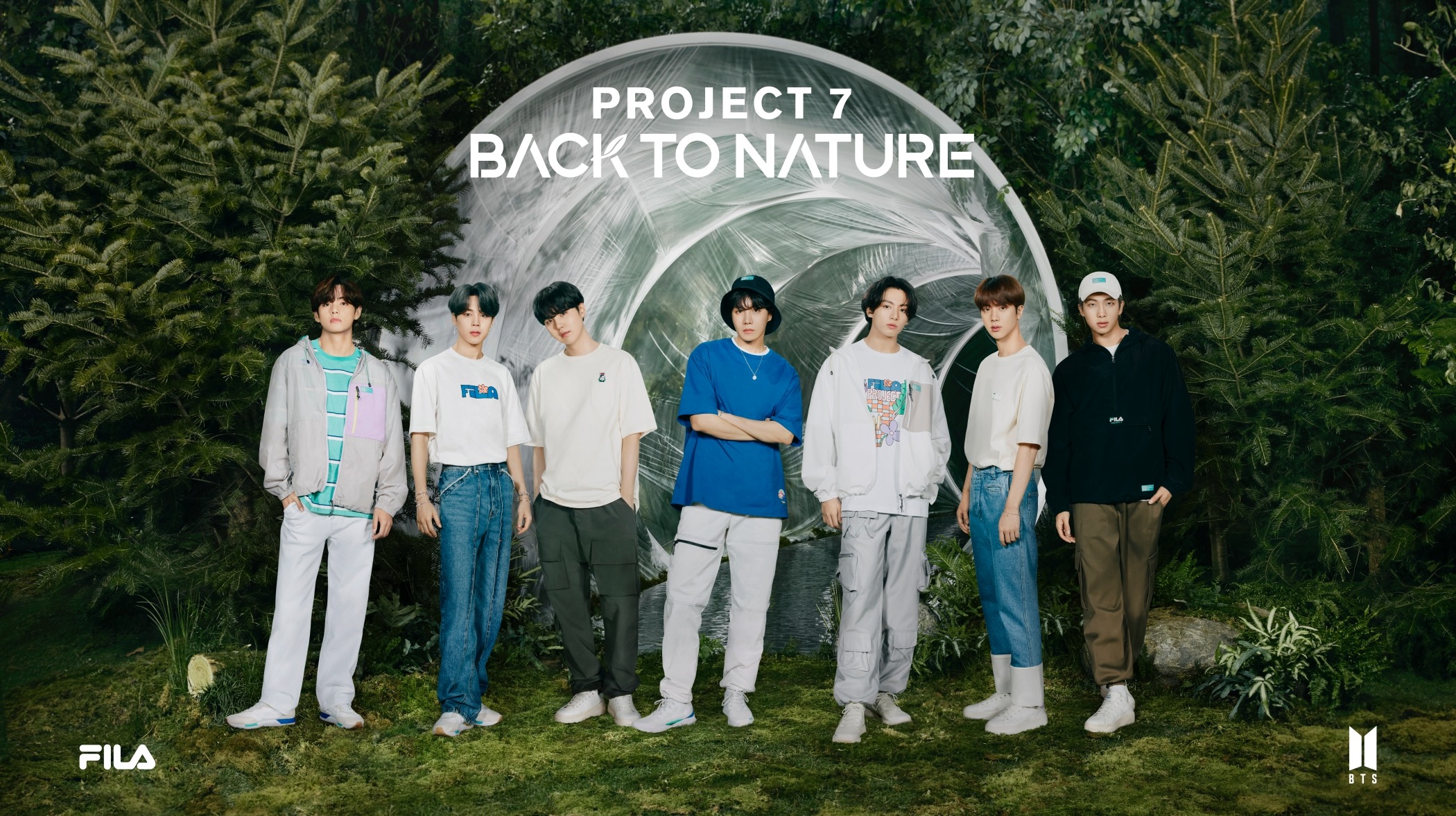This image features the globally renowned Korean boy band BTS, standing in front of a lush, pine-filled forest, creating a serene natural backdrop of vibrant green grass. The band, consisting of seven members, is dressed in FILA streetwear, showcasing a variety of outfits including sweatshirts, t-shirts, jeans, and gray pants, paired with white FILA sneakers. The scene is part of an advertisement campaign titled "Project 7: Back to Nature," aimed at promoting FILA clothing. The text "Project 7 Back to Nature" is displayed prominently at the top of the image, and the FILA logo is featured on the left-hand side in white. Additionally, the BTS logo is situated in the lower right-hand corner, confirming the band's collaboration with the brand. The overall setting and attire emphasize a return to nature, despite the somewhat forced appearance of the young men in the photo.